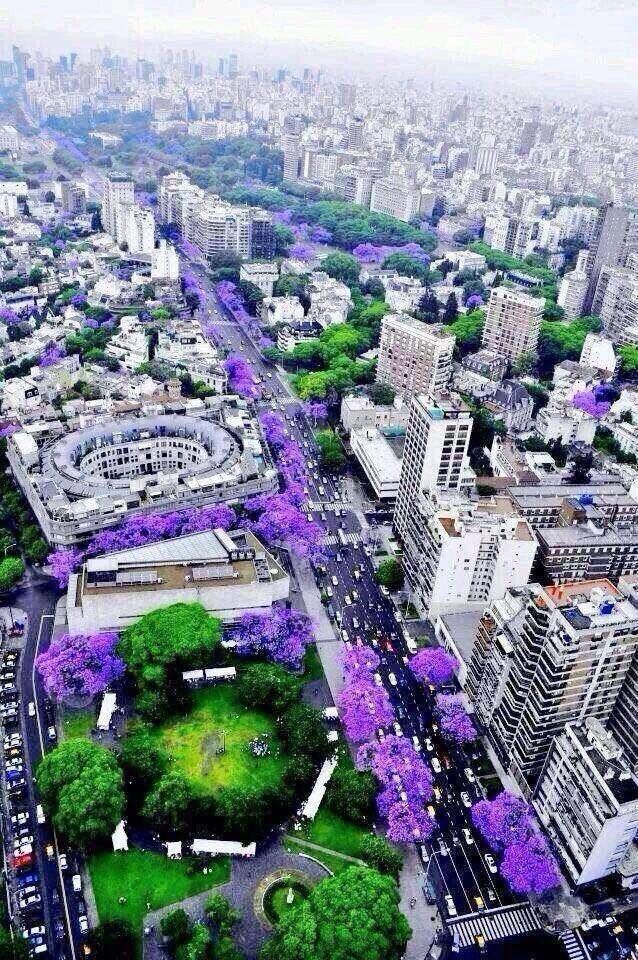The image captures a stunning aerial, panoramic view of a bustling cityscape from a high altitude. Dominated by a mix of residential and commercial buildings, including towering skyscrapers and apartment complexes, the scene is a testament to urban density. Running through the middle of the city is a newly painted six-lane highway, flanked by cars in motion.

Interspersed throughout the urban expanse are abundant patches of greenery, with trees resembling green broccoli florets creating a refreshing, verdant contrast against the concrete landscape. Particularly striking are the numerous bushes and street trees adorned with vibrant lavender-purple flowers, suggestive of a blooming spring season. These bursts of color punctuate the city, injecting life and variety amidst the architectural sprawl.

One notable building stands out with its unique design—an apartment complex featuring a large, dome-like courtyard in its center, adding an element of architectural intrigue. As the view extends towards the horizon, the clarity diminishes slightly, with distant buildings appearing blurrier against a backdrop of low-hanging clouds. This expansive, rectangular shot encapsulates a moment of serene beauty within the bustling city.